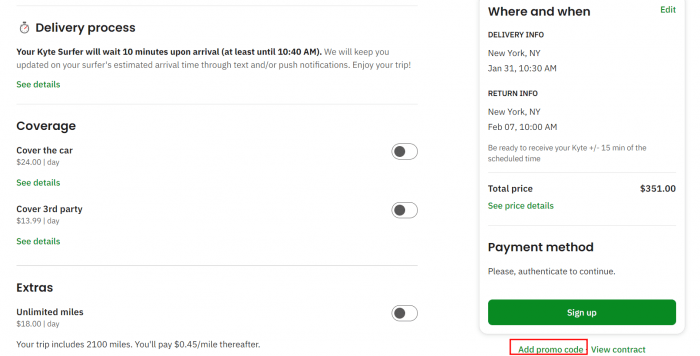**Caption:**

This detailed image appears to be a screenshot of an online booking page for a kite-surfing delivery service. In the upper left-hand corner, there is a "Delivery Process" section accompanied by a clock icon. The text specifies that your kite surfer will wait for 10 minutes upon arrival, until at least 10:40 AM. The service promises to keep customers updated on the arrival time through text and push notifications. There is a green "See Details" link below this text.

Next, there's a coverage section for optional add-ons with two sliders. One is for covering the car ($24 per day), and the other for third-party coverage ($13.99 per day). Both sliders are currently off, with green "See Details" links underneath.

There's an "Extras" section offering unlimited miles for an additional $18 per day, but this slider is also off. The trip includes 200 miles, with an extra charge of $0.45 per mile thereafter.

On the right, the "Where and When" section can be edited using the green "Edit" link. Delivery information lists New York, NY, on January 31st at 10:30 AM, and return info lists New York, NY, on February 7th at 10:00 AM, with a note to be ready to receive your kite within 15 minutes of the scheduled time. The total price is $351, with a green "See Price Details" link underneath.

Below this section is the payment method area, requiring authentication to continue. There’s a prominent green "Sign-Up" button with white text. Additional options include adding a promo code and viewing the contract. A red rectangular outline highlights the "Add Promo Code" section at the lower right-hand corner of the image.